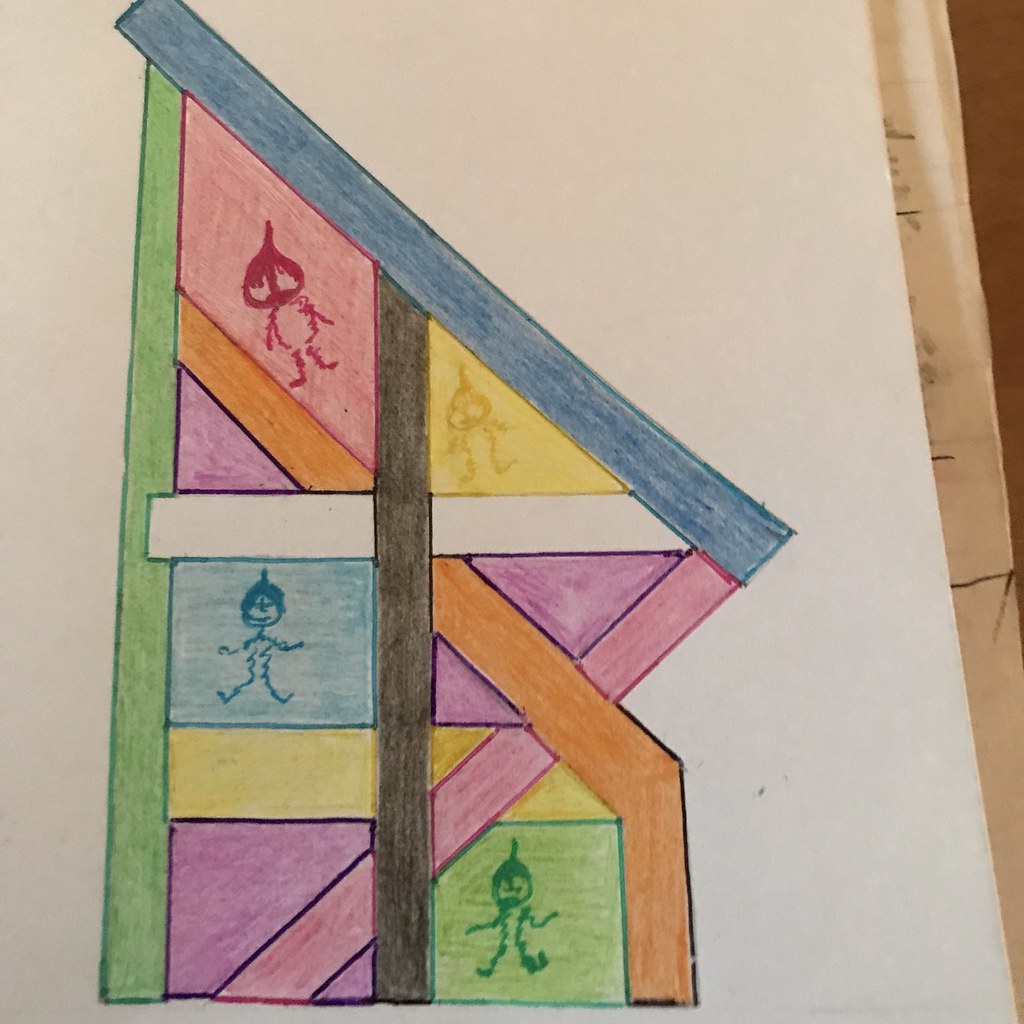The image showcases a drawing on a piece of white paper, which partially overlaps another piece of colored paper on the right, revealing a wedge of brown color underneath that suggests a tabletop surface. The drawing, likely created with markers, features an abstract depiction of a building composed of multiple rectangles oriented both vertically and horizontally, with some positioned diagonally. Within the intersections of these rectangles, there are smaller squares, each containing a stick figure. The figures are meticulously colored to match the hue of their respective squares, but in a darker shade. The vibrant palette includes green, blue, red, yellow, orange, and white, adding a dynamic and lively element to the piece.